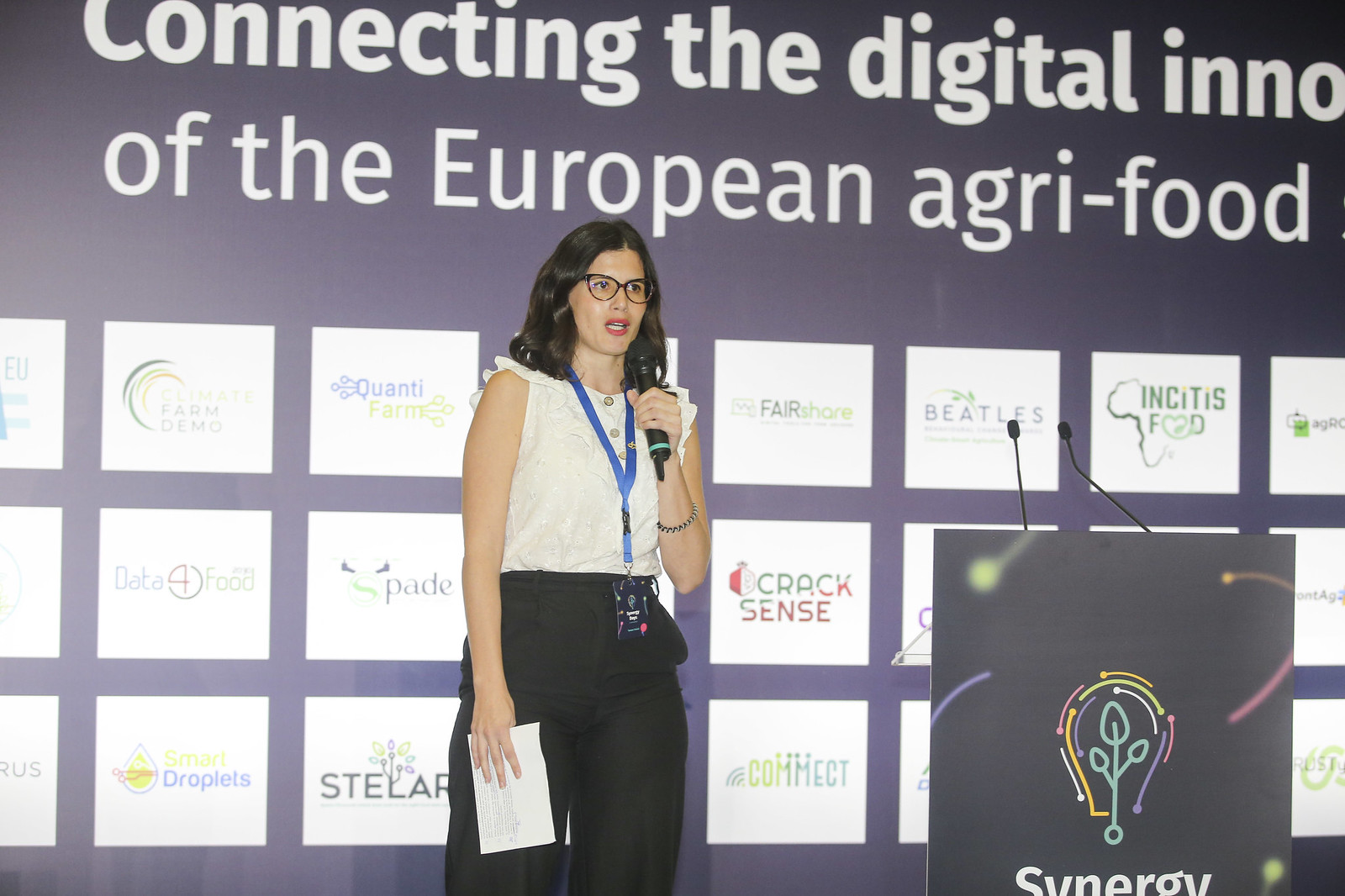In this horizontally oriented photograph, a woman stands at the center, presenting at an event. She wears a white sleeveless top, black pants, and a blue name ID around her neck, accessorized with a bracelet. Her shoulder-length dark hair frames her face, and she wears glasses with a cat-eye shape. She speaks into a microphone held in her left hand, while holding a piece of paper in her right, which rests near her knees. To her right stands a black podium with two microphones and a unique design featuring a multicolored light bulb with a plant-like filament. Below this design, the word "Synergy" is prominently displayed. Behind her, a violet backdrop displays the partially visible title "Connecting the Digital [something] of the European agri-food." The wall is adorned with white tiles, each showcasing various company logos and names, including Farm Demo, Data for Food, Smart Droplets, Stellar, Spade, Quantifarm, Fair Share, Cracksense, Connect, Beatless, and Insight is Food.